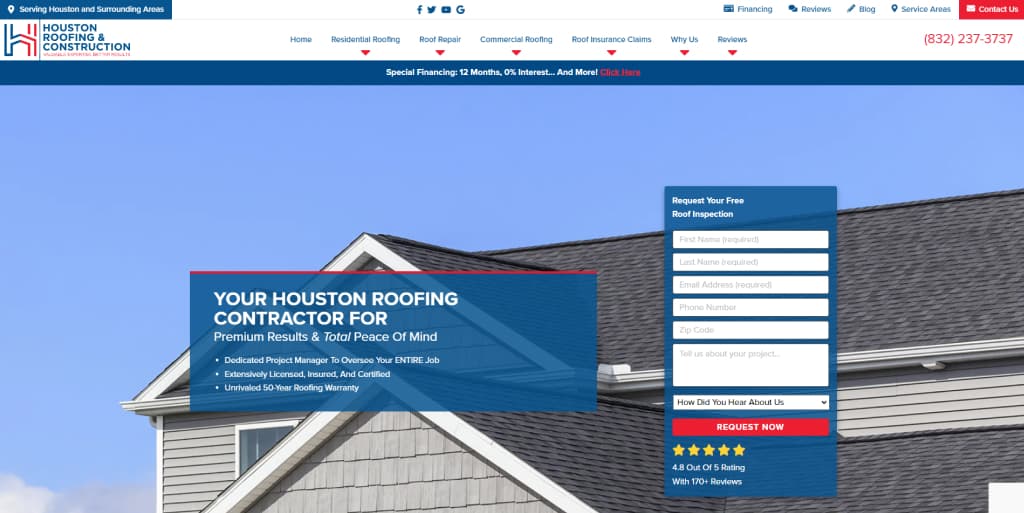The website for Houston Roofing and Construction features a comprehensive layout designed for user convenience and accessibility. The top left corner displays the company's logo with the words "Houston Roofing and Construction," establishing brand identity. At the very top of the page, social media icons for Facebook, Twitter, LinkedIn, and Google are neatly arranged, followed by essential hyperlinks for financing, reviews, blog, service area, and a ‘Contact Us’ link, which is accompanied by the phone number 832-237-3737.

Centered at the top of the webpage, you’ll find navigation links including Home, Residential Roofing, Roof Repair, Commercial Roofing, Roof Insurance Claims, Why Us, and Reviews, allowing easy access to various sections of the site. Below these links is a promotional banner that reads "Special Financing: 12 Months, 0% Interest" with a clickable "Click Here" button.

In the body of the page, there's a visually appealing background featuring a gray house prominently displaying its roof. Overlaying this background are two distinct informational boxes. On the left, a blue box contains bold white text stating, "Your Houston Roofing Contractor for Premium Results and Total Peace of Mind." It details the company’s offerings, including a dedicated project manager to oversee each job, extensive licensing and certification, and an unrivaled 50-year roofing warranty.

To the right, another box prompts visitors to "Request Your Free Roof Inspection." This form asks for the visitor's first name, last name, email address, phone number, zip code, and project details, along with a field asking how the visitor heard about the company. A prominent red button labeled "Request Now" facilitates the submission of this form. Below the button, five yellow stars are displayed, indicating a customer rating of 4.8 out of 5, with over 170 reviews. 

This detailed and intuitive design ensures users can easily navigate the site and access critical information seamlessly.